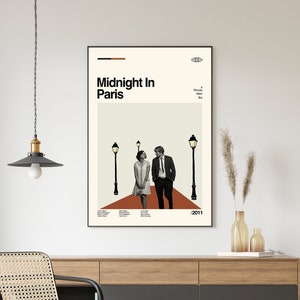In a modern office area, a framed movie poster for "Midnight in Paris" hangs prominently on an off-white wall. The minimalistic poster, boasting a thin black frame, features the title "Midnight in Paris" in bold letters extending along a red street, accompanied by three street lamps. The main characters, including Owen Wilson, walk along this stylized path. Positioned above a wooden desk with a mesh-backed chair and metal sidebars, the scene is complemented by a classic chain-hung lamp. Additional details include two small glass containers filled with wheat and a book on the desk, adding to the room’s decorative elements.